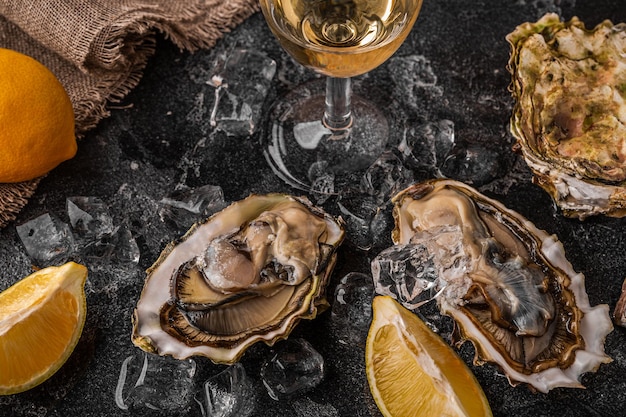In the image, we see what appears to be a variety of shellfish, possibly clams or oysters, arranged on a black, graphite-textured table. The scene is lit from the left, illuminating the stony texture of the table which is covered in partially melted ice. At the bottom of the image, two opened shellfish shells lie next to a couple of lemon slices, amidst the icy spread. Above them, slightly to the left, a wine glass filled with white wine stands, suggesting a top-down side view perspective. To the top left, there’s a piece of frayed cotton or burlap fabric with a whole lemon resting on it. On the right side, there is another large shellfish shell completing the arrangement.